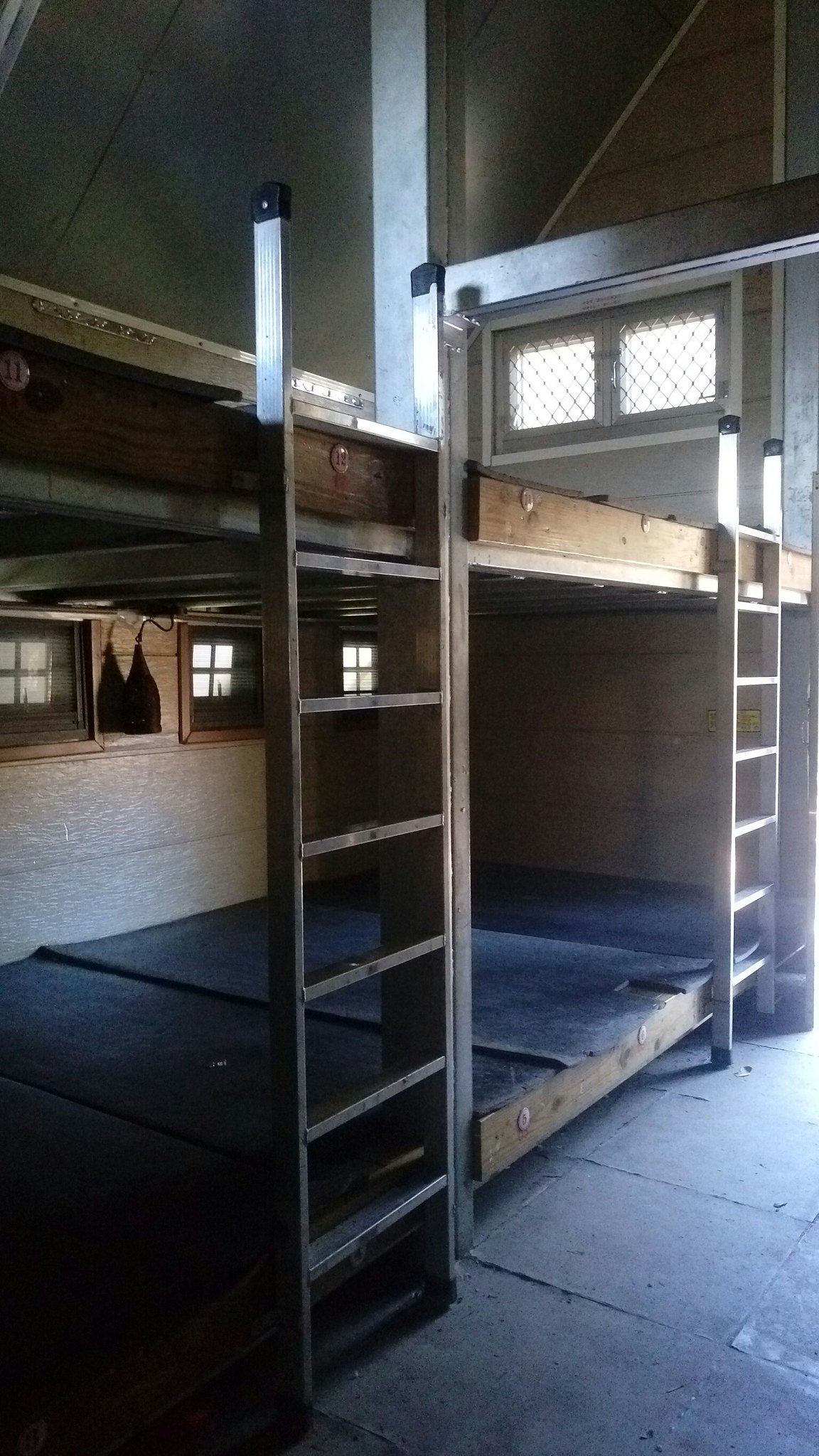The photograph depicts a stark, communal bunk room featuring a row of closely positioned wooden bunk beds, accommodating three individuals per level. Intricately arranged, the lower and upper bunks are connected by makeshift ladders resembling segmented aluminum stepladders, hinting at their potential for extension. Each bunk is topped with thin, blue rubber mats or foam pieces, cut meticulously to fit around the ladders. The room is minimally furnished, with a bare concrete floor adding to the austere atmosphere. Light filters in through a large, open doorway, and a small window with chain-link vents or burglar bars is situated on the far right, further suggesting a highly secured environment. The overall setup, with its sparse amenities and utilitarian design, evokes the harsh living conditions reminiscent of prison camps or makeshift shelters.